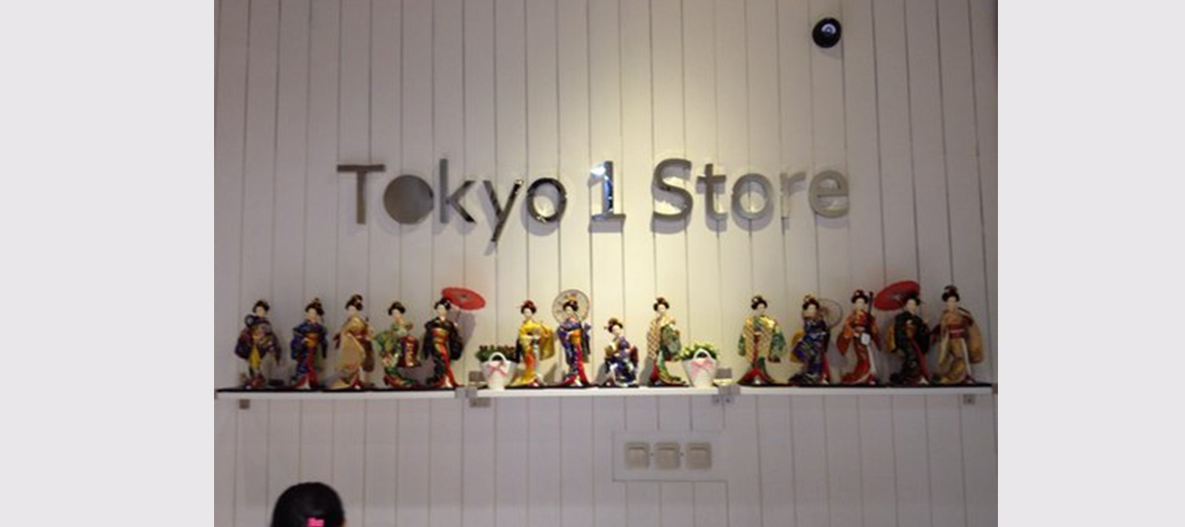This horizontal photograph features a centrally positioned white wall adorned with thin black vertical lines. The wall is flanked by vertical light grey bars on both the left and right sides, each occupying roughly one-fifth of the image's width. At the top-right corner of the wall, a small, dome-shaped security camera is subtly visible. Prominently displayed on the wall are metallic, shiny silver letters spelling out "Tokyo One Store." Below this text, a wooden shelf holds approximately 15 intricately decorated geisha dolls, each around a foot high and dressed in traditional Japanese kimonos. Some of these dolls hold delicate umbrellas. Beneath the shelf, light switches are installed on the wall, and in the bottom-left corner, part of a human head is slightly visible.